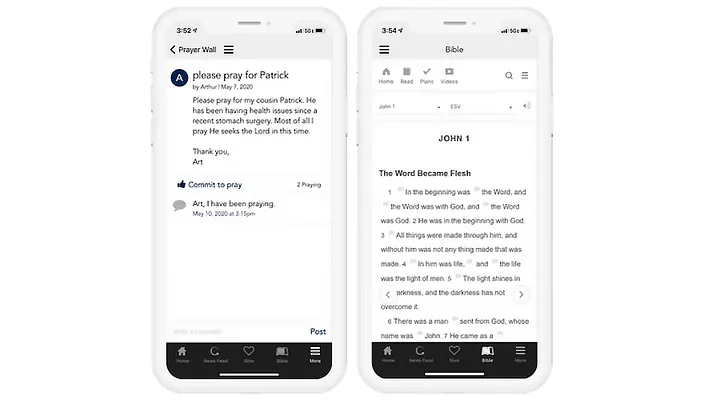This image is a side-by-side screenshot featuring a comment section and a passage from the Bible, all set against a white background. 

On the left side, the screenshot shows a mobile phone interface with a top status bar indicating a location of 352, full cell signal, 5GE network, and a full battery icon. Below that, there is a back arrow followed by the words "Prayer Wall" and a hamburger menu icon, all in black. Within the content area, a prayer request reads: 

"A with a circle. Please pray for Patrick by Arthur, May 7th, 2020. Please pray for my cousin Patrick. He has been having health issues since a recent stomach surgery. Most of all, I pray he seeks the Lord in this time. Thank you, Art."

Below the request, options to "Comment" or "Commit to Pray" are shown alongside a thumbs-up icon. There is also a conversation bubble icon with a response that states: 

"To praying. Art, I have been praying."

On the right side of the image, another phone screen displays the Bible app interface. The top menu shows the word "Bible" with six different menu icons. Below that, the passage from John 1 in the English Standard Version (ESV) is displayed:

"John 1: The Word Became Flesh." (bold and centered)

"In the beginning was the Word, and the Word was with God, and the Word was God. He was in the beginning with God. All things were made through him, and without him was not anything made that was made. In him was life, and the life was the light of men. The light shines in the darkness, and the darkness has not overcome it. There was a man sent from God, whose name was John. He came as a witness..." (unbolded and in black text)

At the bottom of both phone screens, the standard menu options for the phone's interface are visible on the left and right phones respectively.